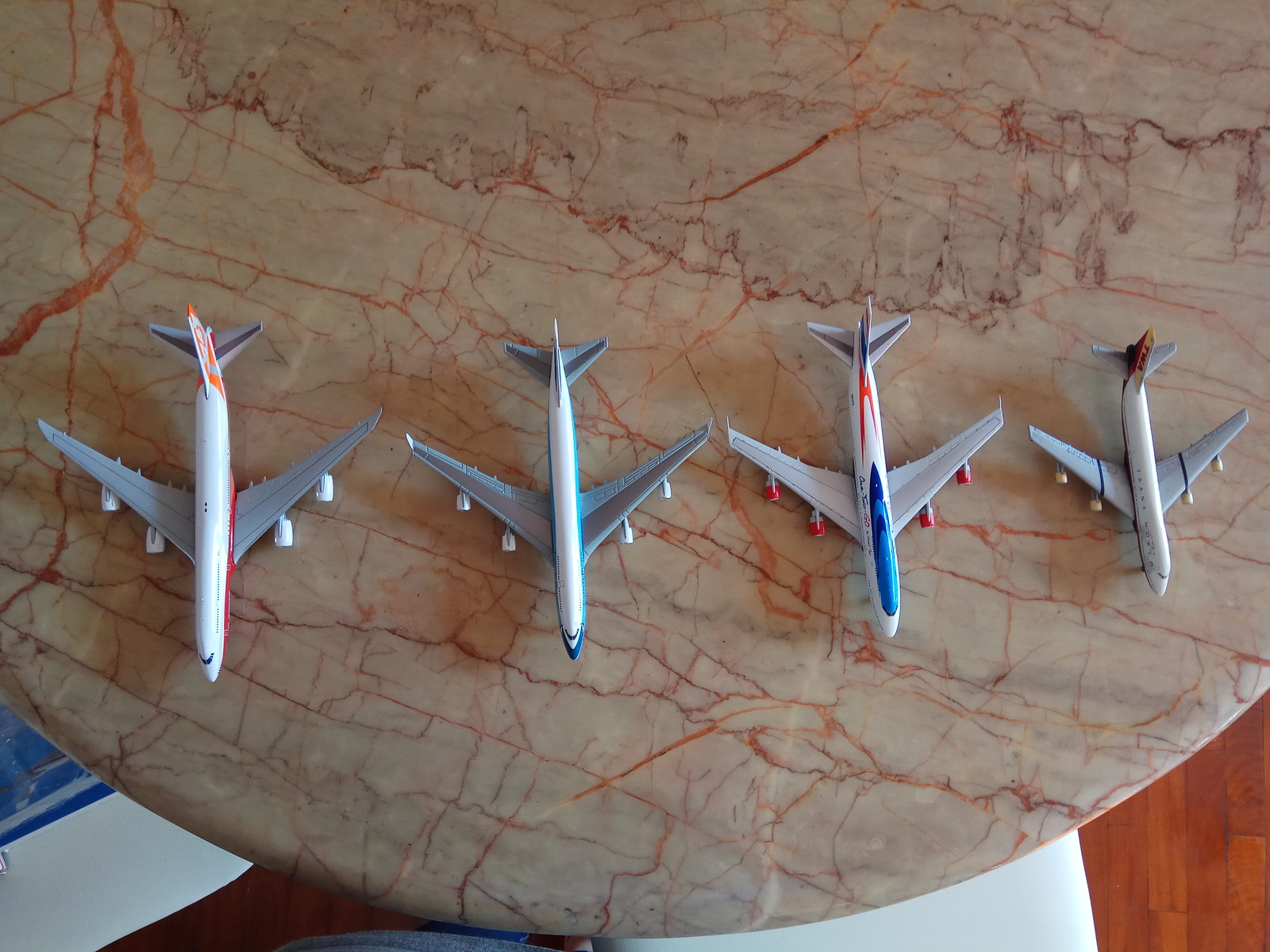The photograph, taken indoors, features a round coffee table with a beige, cream, and reddish marble-like design. The table stands on a floor with varying shades of reddish wood, and in the background, a couple of white chair seats are visible. On the tabletop, there are four model airplanes, all four-engine jets with swept-back wings and a triangular tail configuration.

1. The airplane on the far right is the smallest, predominantly white with a red stripe down the tail.
2. Next to it, the second plane exhibits a grey and blue design. It has a blue nose tip, grey stripes on its wings, and additional red markings around the fuselage and tail.
3. The third aircraft, more detailed, features a light blue nose and a mix of blue and grey on the wings. Its tail includes some blue and likely Asian characters, with a red stripe running on the side.
4. The fourth plane, on the far left, sports a prominent red stripe down its fuselage, with orange or red designs on the tail and hints of grey on the wings.

In the background, the floor's various tan shades and the blue and white elements add to the intricate setting.